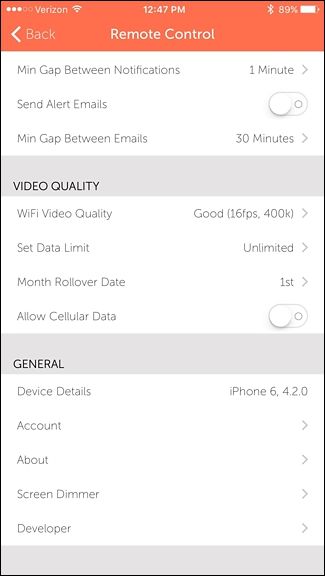In this detailed screenshot from an app, we are greeted with a top-center header labeled "Remote Control," accompanied by a back button on its left. Below this header, we encounter various settings sections. 

The first section states "Min Gap Between Notifications," which is set to 1 minute. The "Send Alert Emails" option in the section is turned off, while the "Min Gap Between Emails" is set to 30 minutes. 

Following this, we move to the "Video Quality" section. It indicates that the Wi-Fi video quality is set to "Good," with specifications of 16 FPS and a bitrate of 400K. The setting "Set Data Limit" is marked as "Unlimited," and the "Month Rollover Date" is set to the first of each month. The "Allow Cellular Data" option is turned off.

The final section is labeled "General." This area provides comprehensive information and includes options such as "Device Details" (iPhone 6, version 4.2.0), "Account," "About," "Screen Dimmer," and "Developer." Each of these options has a right-pointing arrow next to it, indicating that they are expandable and likely link to additional settings or information on separate tabs.